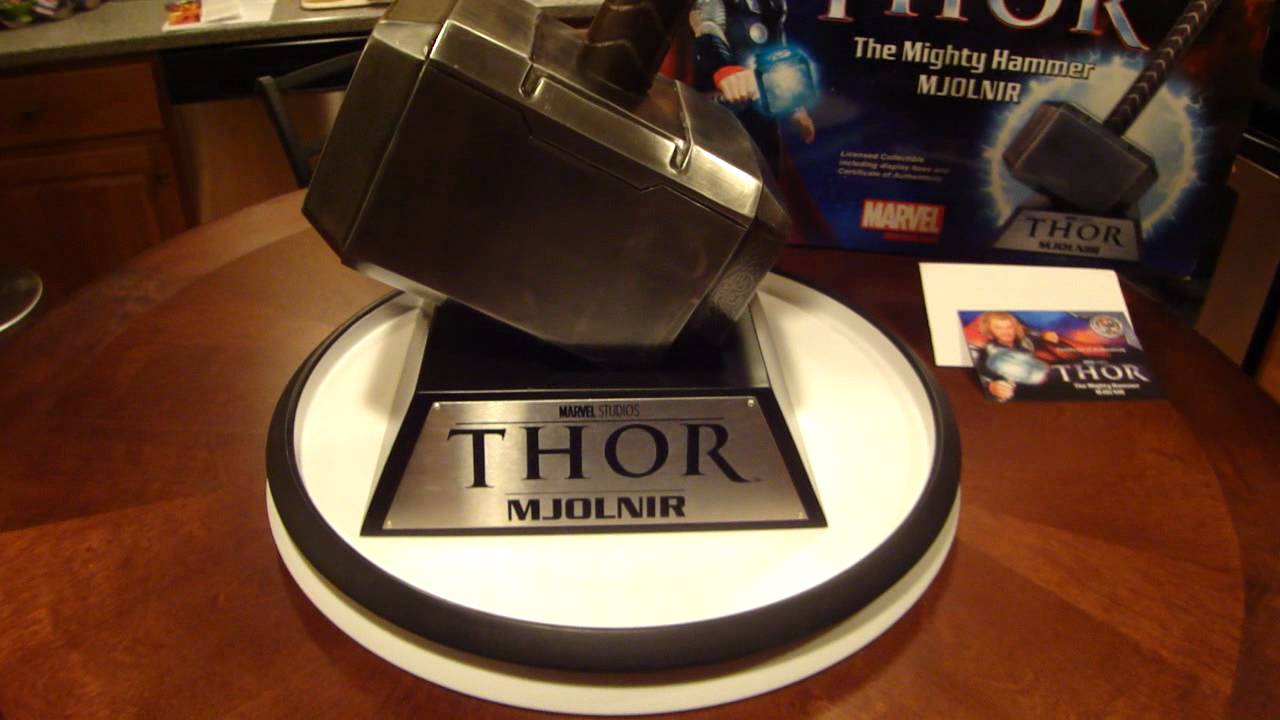In what appears to be a home setting, possibly a kitchen or an office, we see a detailed display of a collector's item: a replica of Thor's hammer, Mjolnir, from Marvel Studios. The hammer is placed elegantly on a rich, reddish-brown round wooden table. The table also supports a flat, circular display stand, which is white with a black trim around the edge. In the center of this platform, there is a black plaque with a silver plate inscribed with "Marvel Studios, Thor, Mjolnir."

The hammer itself, although it appears metallic, is tilted with the right side angled down into the stand and the left side raised. You can observe the silver square head of the hammer, and part of its handle with scale-like ridges in brown.

In the background, the black box for the hammer is visible, partly cut off but displaying distinct features. On the box, Thor is depicted holding Mjolnir, wearing his blue suit with large silver circles and a silver arm band. The box features text that reads "The Mighty Hammer, Mjolnir," along with text and imagery consistent with Marvel branding. Additionally, there is a piece of white paper with an image of Thor holding the hammer, slightly tilted and resting in front of the box. The overall scene captures the essence of a prized collector's display in a cozy, personal space.